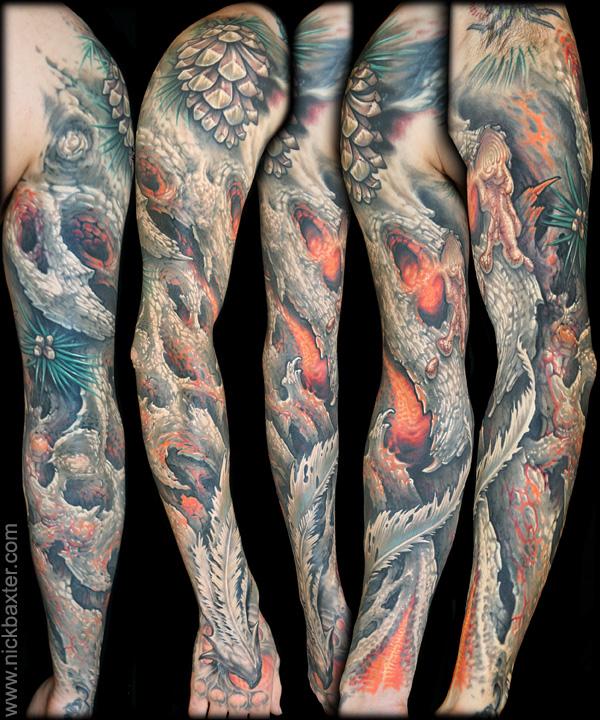The image is a composite of five photographs capturing a man's intricately tattooed arm from various angles. The tattoo, which covers the entire arm from the knuckles to the shoulder, is a vividly colored full sleeve. It integrates various elements and hues, creating a complex and multi-layered design. Predominantly, the tattoo features a mix of black, red, orange, white, and brown textures, which together add depth and complexity.

Prominently, the design includes an intricate depiction of a dragon with a pointed beak and feathers that cascade from its neck, transitioning smoothly around the arm. The themes are predominantly naturalistic, with elements such as a large pine cone with accompanying pine needles near the shoulder, feathers, and a swirling background that alternates between resembling clouds or rocks, present throughout the tattoo. These natural elements are interwoven with fiery, lava-like patterns primarily displayed on the inner arm. 

The tattoo also integrates sections of greenish-gray, darker green, and golden-yellow tones. The top of the arm exhibits textures reminiscent of tree bark and reddish fiery swirls. Furthermore, in some sections, a goldish liquid appears to be oozing from the design, adding to its layered intricacy. Overall, the tattoo is a masterful blend of natural and fantasy elements, executed in a range of colors and textures, creating a visually striking and encompassing sleeve. The images are set against a black background, with the website www.nickbaxter.com inscribed vertically on the left, presumably attributed to the photographer or artist.